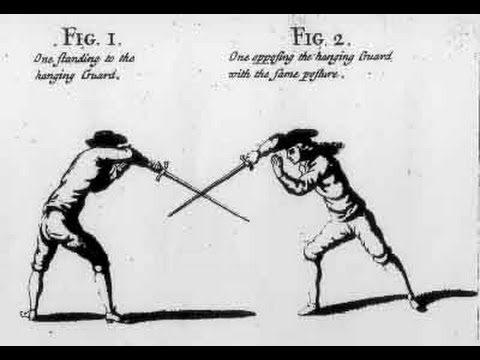This black-and-white sketch, reminiscent of an older Renaissance or possibly 1800s-1900s style, captures a dramatic scene of two men engaged in a fencing duel. The illustration is labeled with "Fig 1" in the upper left corner and "Fig 2" in the upper right corner, with faintly readable captions below each figure. Fig 1 is described as "One Flanking to the Hanging Guard," while Fig 2 reads "One Appealing the Hanging Guard with the Flame," though the final word remains unclear due to the cursive font. Both men are intensely focused on each other, their arms raised, and their swords crossed in a defensive stance. They wear stereotypical fencing attire: long-sleeve white shirts, knickers ending just below the knees, and long socks, all rendered in a grayish white. Completing their period look, each man dons a black fedora hat, and one has long hair. Their long shadows stretch across the ground, adding depth to the scene.